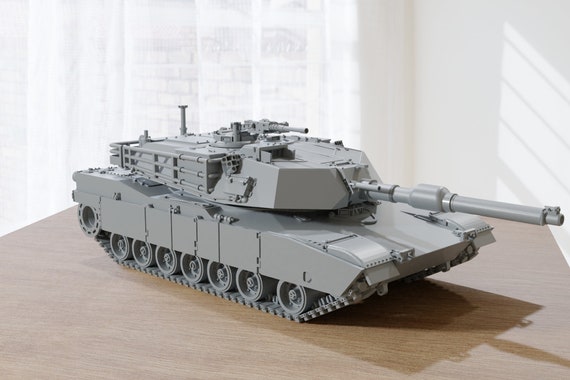This image features a detailed model of a modern M1A Abrams tank, predominantly dark gray in color with some hints of olive green. The tank is positioned on a light wooden table, casting distinct shadows toward the bottom right due to a light source originating from the back top left corner. The model showcases a variety of features, such as numerous square sections of armor above the tracks, and intricate fencing along the backside, likely designed to represent anti-rocket protection measures. Two flaps are visible near the top edges of the tank's tracks, possibly simulating additional lighting or protective features.

The tank is orientated with its cannon and turret pointed to the right, and it's equipped with a machine gun mounted on top. Each side of the tank features nine wheels, crucial for its mobility. Behind the tank, the background consists of a white, somewhat translucent curtain through which a brick wall can be faintly seen, accompanied by a white-painted window and trim on the left, and plain white walls on the right. This combination of detailed elements and realistic environments showcases the craftsmanship and attention to detail in the model tank.